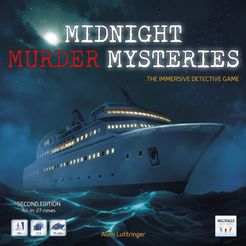The image is a square front cover of a game, overall designed to depict a mysterious nighttime scene. At the top of the cover, in typewriter font, it reads "Midnight Murder Mysteries." "Midnight" and "Mysteries" are in white text, while "Murder" is prominently highlighted in red. Below this title, smaller yellow letters read "The Immersive Detective Game," all in capitals. In the top left corner, the moon breaks through dark blue clouds, casting a silvery light across the scene.

Centered in the image is a large, two-story ship sailing through a rough, choppy sea. The ship is largely dark, with most cabin lights switched on, adding an eerie glow. The reflection of the moonlight on the sea creates a striking contrast against the dark water.

In the bottom left corner, "Second Edition" is displayed in white text. Directly below this, there are three small, indiscernible square images. A name, only partially legible and suspected to be "Lutringer," appears in the center of the lower part of the cover in yellow letters. In the bottom right corner, another light-colored square with unreadable text is visible.